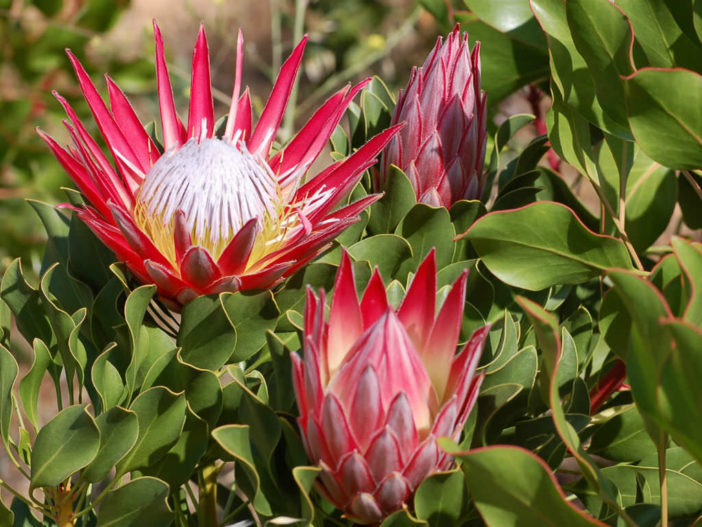This up-close photograph captures a striking and unique group of flowers set against a vibrant backdrop of green foliage. The green leaves are wavy and curly, with beautiful reddish-pink outlines enhancing their bright green color. In the center of the image, three flower blooms or buds are prominently featured. One of the flowers, located to the left, is fully open with long, spiky red petals radiating outwards and a round center that is white with yellow tips. The flower in the front is partially open, revealing its emerging red petals while still maintaining a conical shape. The third flower, situated to the right, remains completely closed, resembling a red pine cone or a dragon fruit in appearance. The detailed red and yellow coloring and the needle-like petals make these blooms exceptionally distinctive and visually captivating.